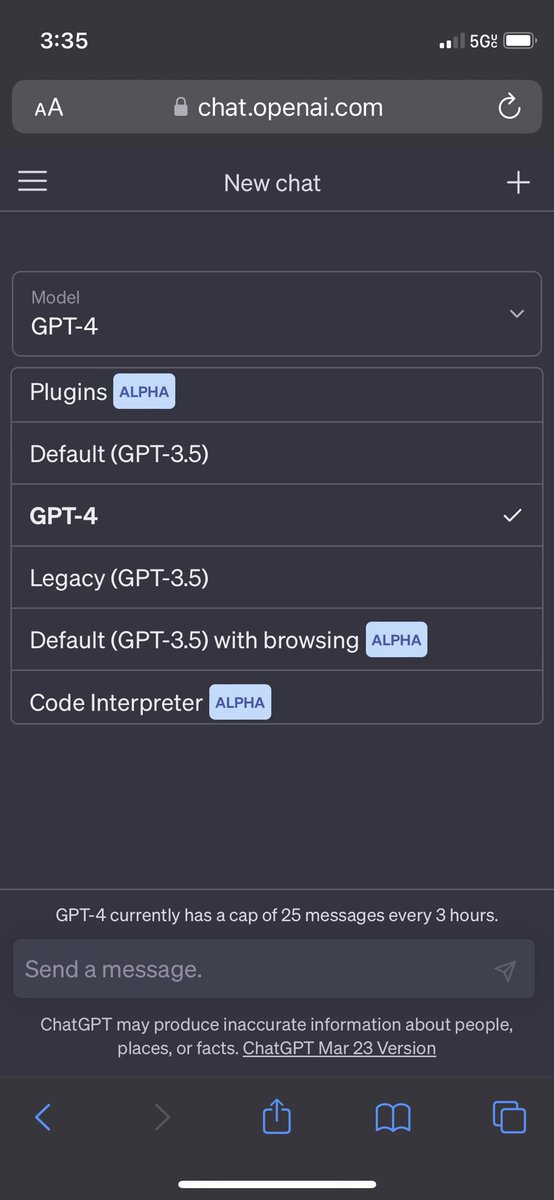This is a detailed, cleaned-up caption:

"A cell phone screenshot displaying the interface of OpenAI's ChatGPT platform. The screenshot, in a rectangular format that is taller than it is wide, features a light black background. At the top of the screen, the status bar shows the time as 3:35 PM in the upper left corner, while the upper right corner displays the signal strength, a nearly full battery icon, and a 5G indicator. Below the status bar, a web address bar contains the URL: chat.openai.com.

Directly beneath the web address bar is a button labeled 'New Chat,' allowing users to initiate a new conversation. The interface then offers a selection of options for the type of chatbot to use, each presented in separate boxes. These options include:

- ChatGPT-4
- Plug-in (marked as Alpha)
- Default (GPT-3.5)
- GPT-4 (Legacy)
- Default (GPT-3.5 with browsing capabilities, marked as Alpha)
- Code Interpreter (marked as Alpha)

At the bottom of the screen, additional text notes that 'GPT-4 currently has a cap of 25 messages every three hours.'

Further down, a message input bar is visible for sending messages. A disclaimer below it cautions, 'ChatGPT may produce inaccurate information about people, places, or facts.' The version of ChatGPT displayed is 'Mar-23 version.'"